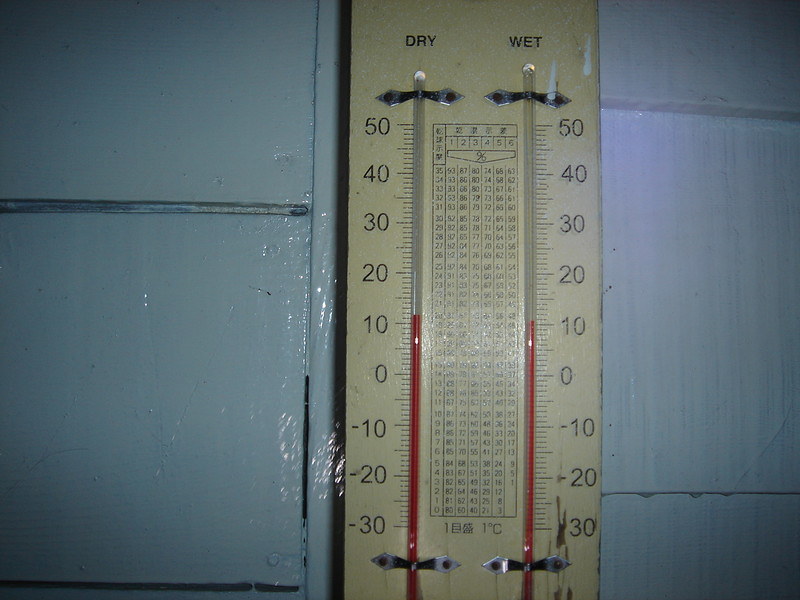This image features a detailed close-up of a dual-thermometer hygrometer mounted on a wall with cream-colored painted paneling. The hygrometer's housing is an off-yellow color. On the left side of the device, the dry thermometer's scale ranges from 50 down to -30 degrees, clearly labelled with major increments: 50, 40, 30, 20, 10, 0, -10, -20, and -30. On the right side, the wet thermometer mirrors the same temperature scale. Centered between the two thermometers is an intricate chart, labelled 1 through 6, alongside percentage signs and various numbers for interpreting humidity levels. Both thermometers contain red liquid, indicating the temperature, with the dry thermometer reading slightly above 10 degrees and the wet thermometer just a fraction below that of the dry thermometer. Sturdy metal clamps secure the glass bulbs of each thermometer firmly onto the device.